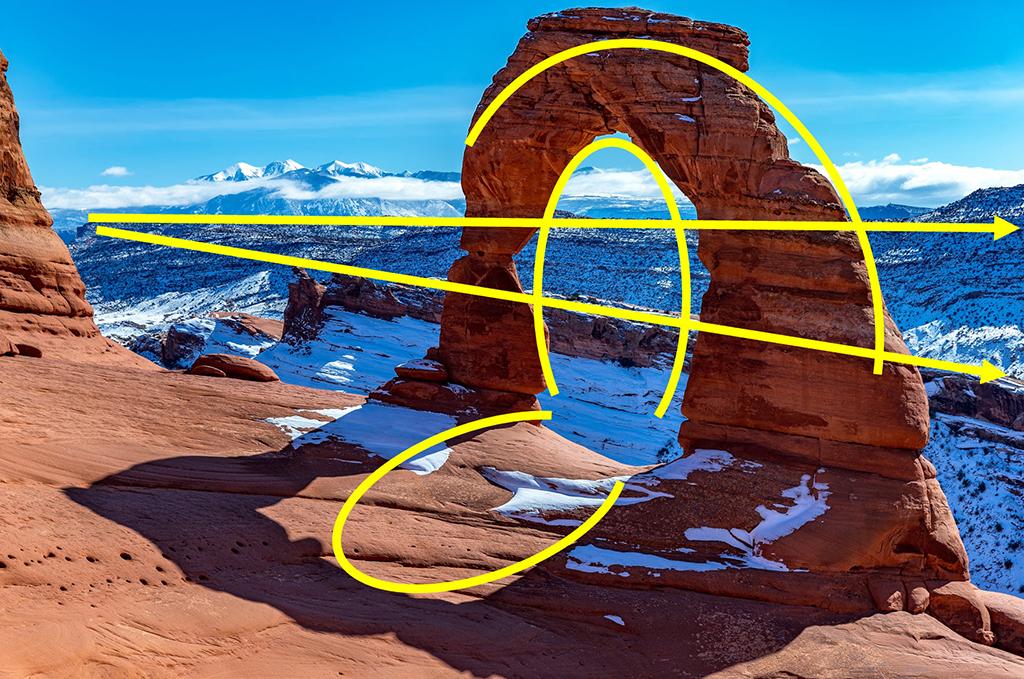In this outdoor scene, a stunning snowy landscape unfolds beneath a clear blue sky with scattered clouds. Dominating the foreground is a striking, naturally formed rock arch crafted from reddish-brown stone. This arch frames a large oval cutout at its center, creating a dramatic window through which the snow-covered hills and distant mountains can be glimpsed. The backdrop showcases snow-covered mountains, adding immense depth to the scenery. The ground immediately surrounding the rock arch has only a light dusting of snow, revealing the rocky terrain beneath.

Superimposed on the image are several yellow lines, indicative of some form of diagram or perspective analysis. A yellow line runs along the top and right side of the arch's cutout. Two straight yellow lines extend across the photo from the left, with an arrow at the end of these lines pointing toward the right side of the screen. Beneath the arch's opening, another yellow line outlines the base, while a semi-oval line is drawn from the opening down to the base of the rock, emphasizing the arch's curvature and dimensions against the snowy backdrop.